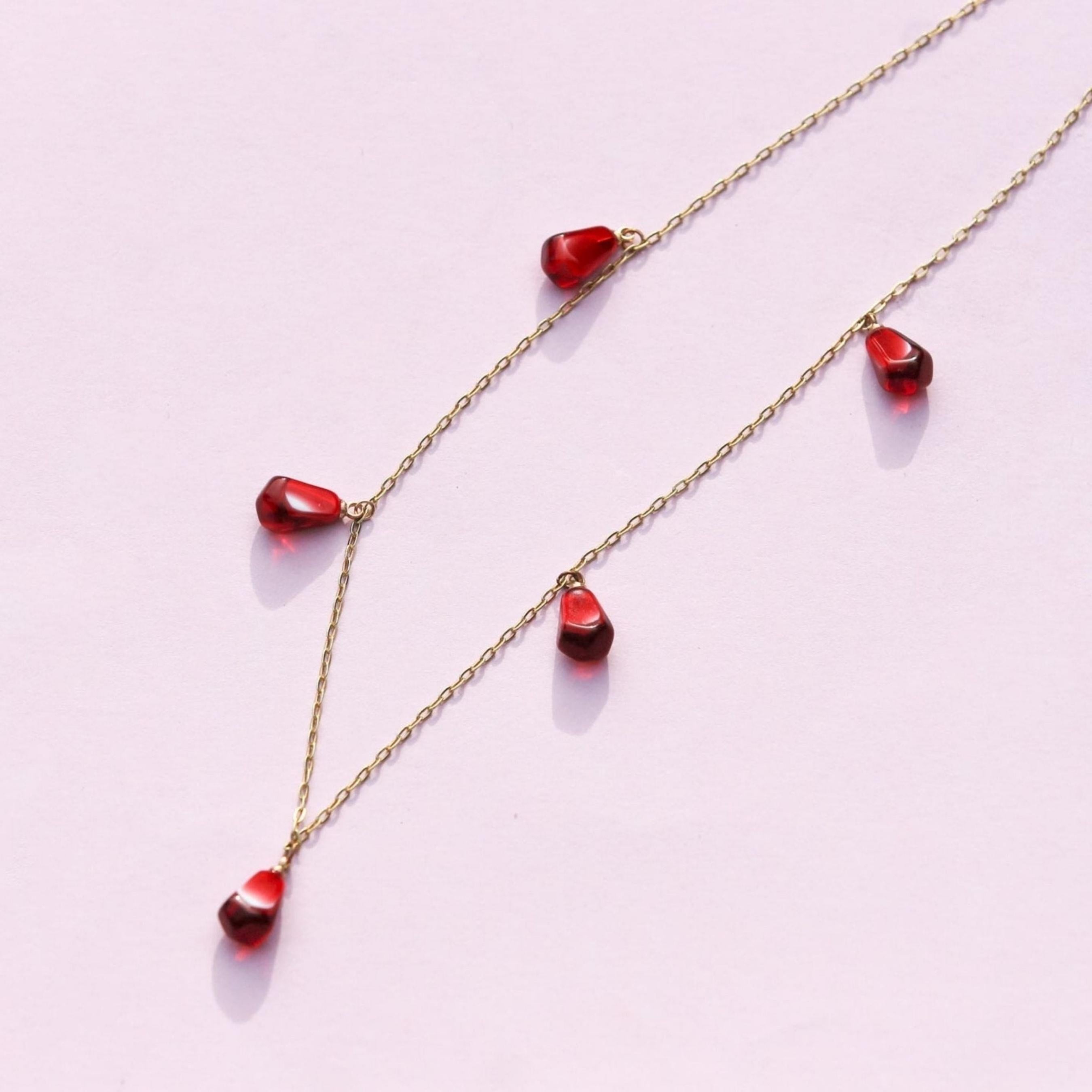The image is a close-up photograph of a delicate gold necklace. The necklace is laid out diagonally on a slightly pink background, with the chain running from the bottom left to the top right. This gold chain features five evenly spaced red gems that resemble pomegranate seeds or blood droplets, adding an elegant yet bold touch. The gems, likely rubies, are small, shiny, and dainty, with light reflecting off their surfaces and casting subtle shadows beneath. These gems are attached to the chain with little gold links, giving the necklace a refined and cohesive appearance perfect for display.